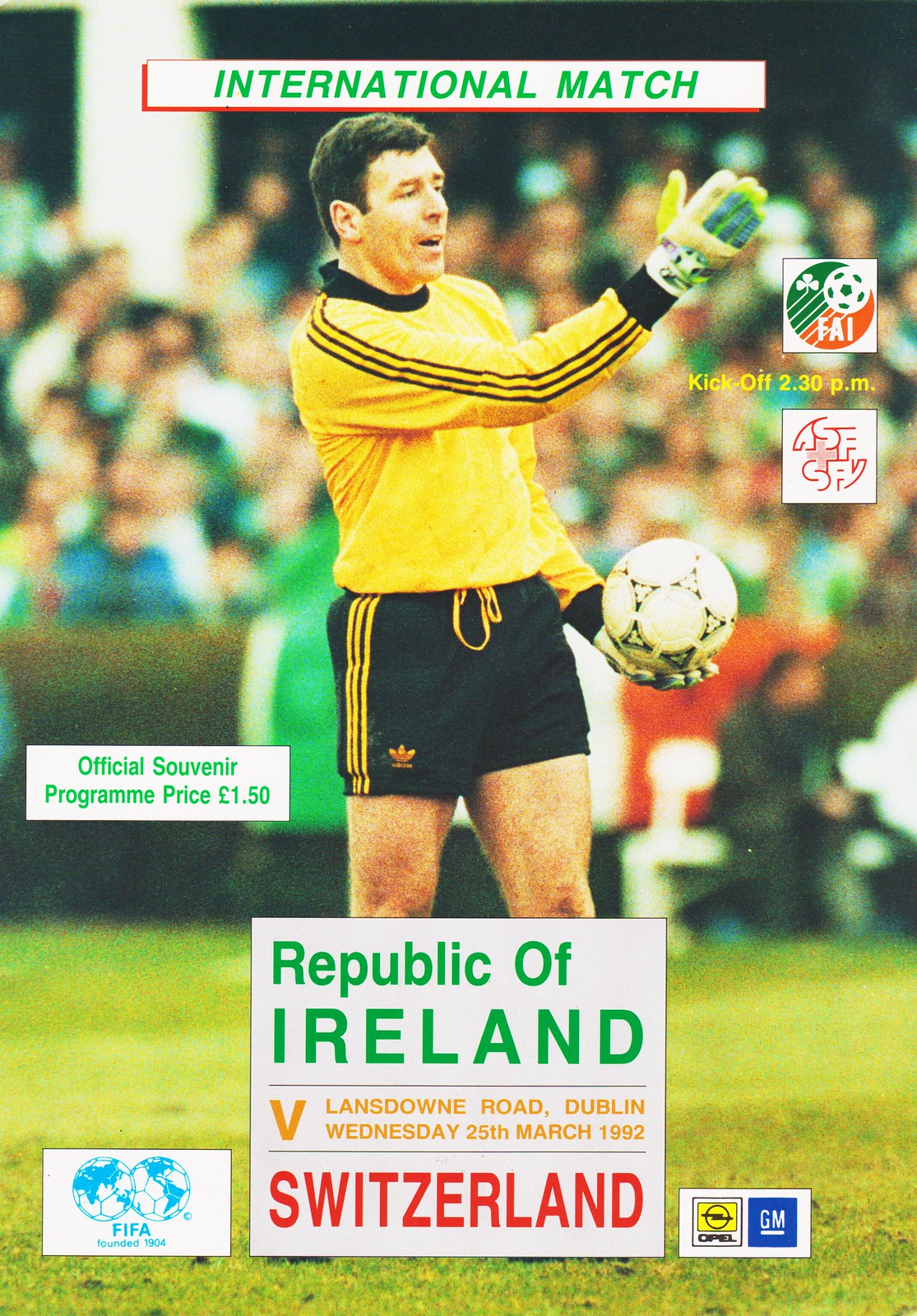This is a photograph of the cover of an official souvenir program priced at one pound fifty pence. Across the top, "International Match" is written in green lettering on a white background framed in red. A man, holding a soccer ball in his left hand and raising his right hand, stands prominently on the cover. He is dressed in a yellow shirt with black stripes, a black collar, and cuffs, paired with black shorts featuring yellow stripes. He also wears yellow and green gloves. Below the man’s knees, the text reads "Republic of Ireland, Lansdowne Road, Dublin, Wednesday 25th March 1992" in green, yellow, and red type against a white background. Flanking him are various logos: to the left is the FIFA logo, and to the right are the Opel and GM logos. Positioned underneath a logo displaying a soccer ball and a three-leaved clover with the letters FAI, is another logo labeled ASF/SFY. In the background, although blurred, the stands and the field are visible.